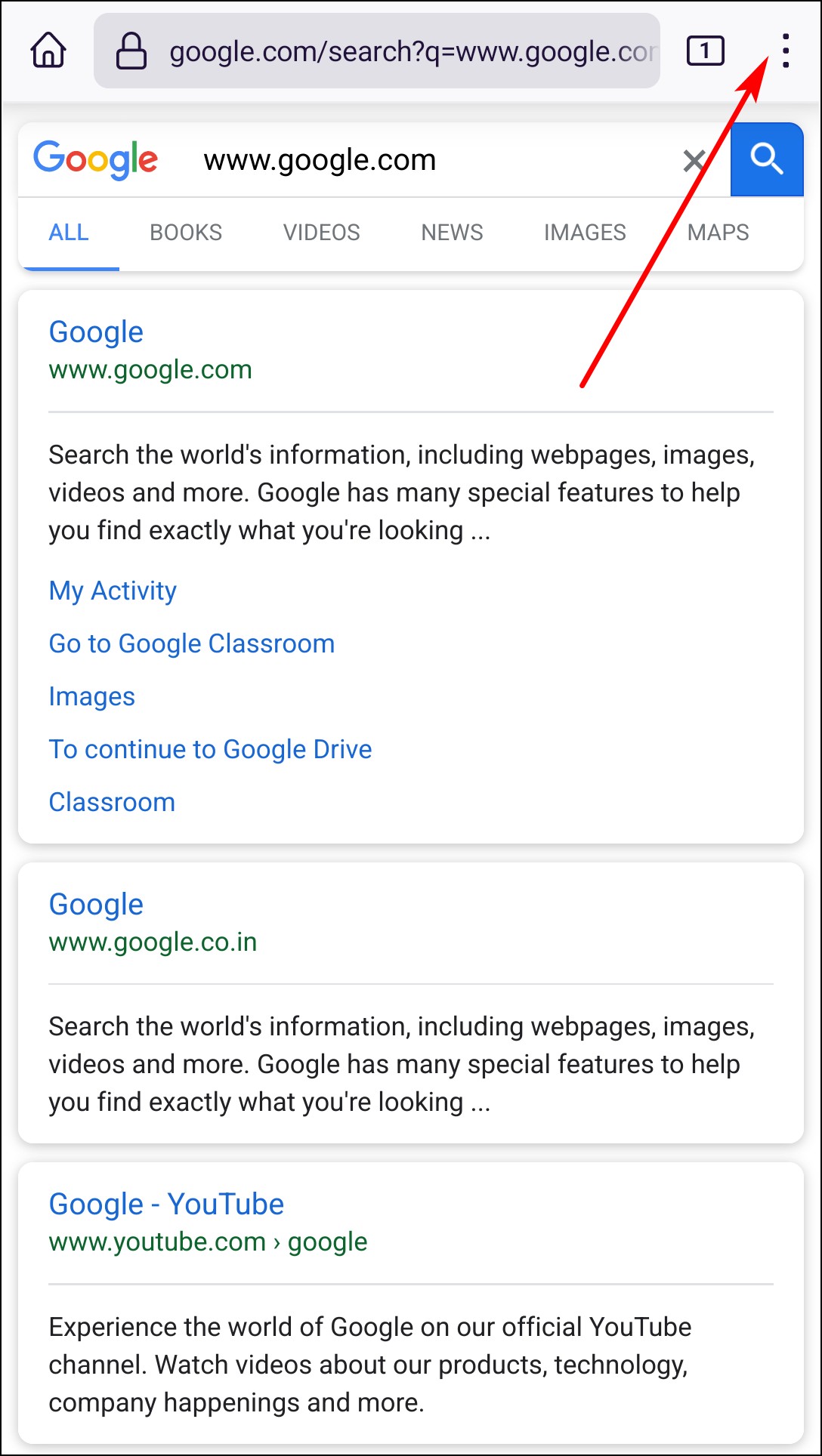The image is a smartphone screenshot of the Google homepage. At the top, the interface is predominantly white with black text and blue links. There is a home icon visible, and the search bar contains the URL "google.com/search." Also notable is a button indicating that one tab is open, alongside a red arrow pointing to a vertical three-dot menu in the upper right corner.

Below this, the familiar Google logo is displayed above the search box, which contains the URL "www.google.com." Adjacent to the search box is an arrow icon for closing it out. Underneath the search box, there are several tabs labeled "All," "Books," "Videos," "News," "Images," and "Maps," with the "All" tab currently active.

Further down, a text description reads: "Google - www.google.com. Search the world's information, including web pages, images, videos, and more. Google has many special features to help you find exactly what you're looking for..." (an ellipsis indicating additional text not fully displayed).

Below this, there are links labeled "My Activity," "Go to Google Classroom," and "Images." Another section follows with a similar format, reiterating the Google domain and functionality: "Google - www.google.com. Search the world's information, including web pages, images, videos, and more. Google has many special features to help you find exactly what you're looking for..."

At the bottom of the screenshot, there is an entry for "Google-YouTube - www.youtube.com," followed by text stating: "Experience the world of Google on your official YouTube channel. Watch videos about our products, technology, company happenings, and more." An arrow icon to the right points forward.

The layout, colors, and icons all contribute to a typical, easily recognizable Google search page setup, providing a clear snapshot of the interface and options available to users.